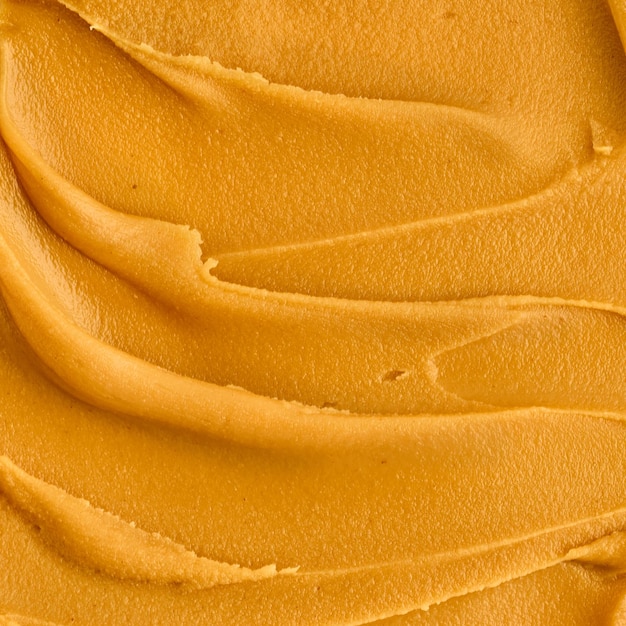This image is a highly detailed, square-shaped close-up of a brownish-orange spread that appears to be peanut butter, although it could potentially be frosting or a similar substance. The photograph captures the texture and color of the spread, which is thick and firm with a grainy appearance and distinct swooping knife marks running from left to right. The knife strokes create little waves that rise and crust at the tops, held in shape rather than dripping like a liquid. Slight shadows form beneath these waves, suggesting a light source shining across the surface, though its exact origin is unknown. The entire frame of the image is filled with this textured spread, giving a detailed and immersive view of its consistency and color.